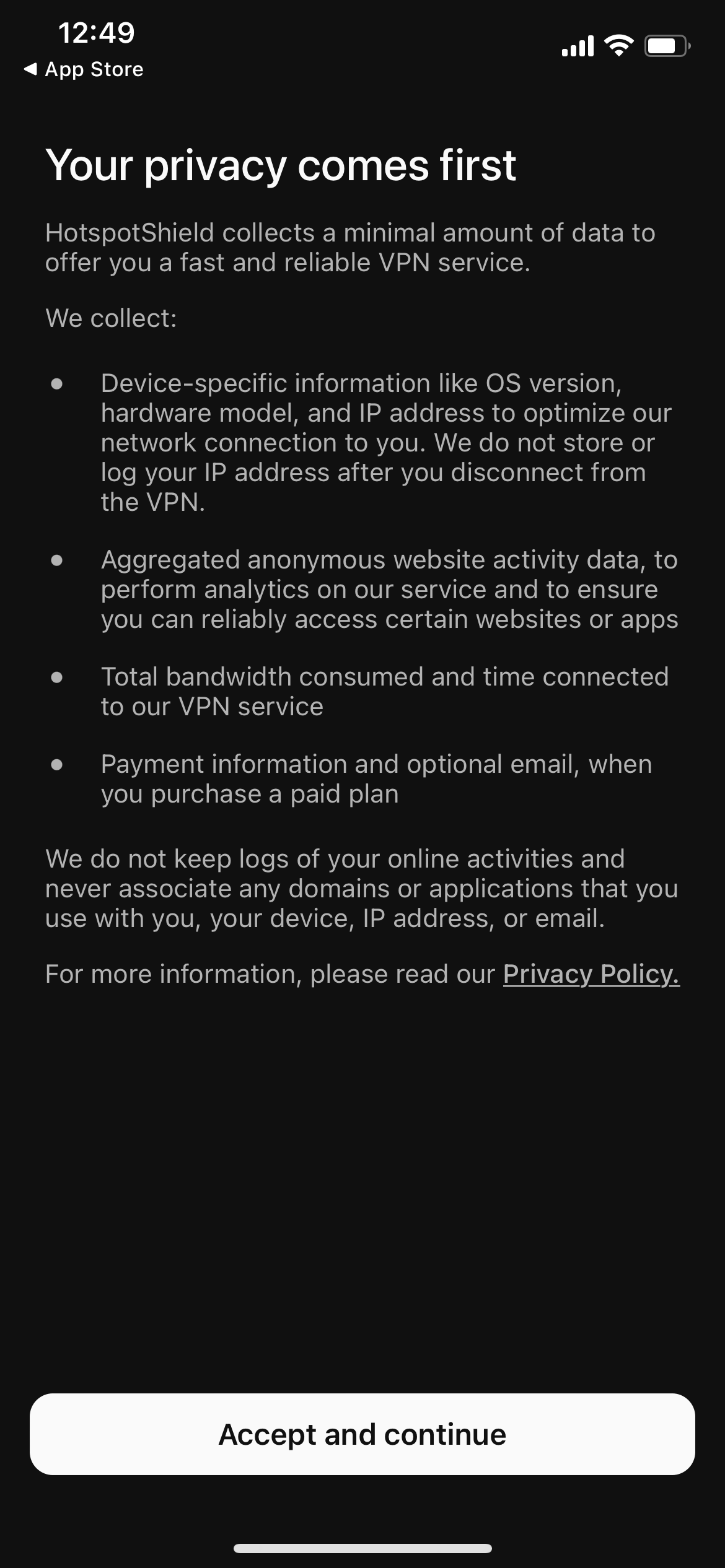This is a detailed screenshot of a mobile device screen displaying the Apple App Store interface. The background is black, giving prominence to the content. 

- **Top Left Corner**: The time displayed is 12:49.
- **Underneath the Top Left Corner**: The title "App Store" is shown, with a left-pointing arrow next to it.

- **Top Right Corner**: Indicators show a battery icon at approximately 80% charge, along with fully active Wi-Fi and Internet connection signals.

- **Main Content**: 

    - **Header**: In bold white letters, it states, "Your Privacy Comes First."
    - **Subheader**: Below, in smaller white text, it reads: "Hotspot Shield collects a minimal amount of data to offer you a fast and reliable VPN service."

    - **Data Collection Details**: A section titled "We Collect" is presented, with four bullet points aligned on the left side. Each bullet point has varying lines of text:
        1. The first bullet point has five lines of information.
        2. The second bullet point contains three lines.
        3. The third has two lines.
        4. The fourth also consists of two lines.

    - **Additional Privacy Information**: Underneath, a statement says, "We do not keep logs of online activities and never associate any domains or applications that you use with your device, IP address or email."

    - **Policy Link**: Further down, it mentions, "For more information, please read our privacy policy." This text is underlined, indicating a clickable link.

- **Action Button**: Near the bottom of the screenshot, there is a large white tab stretching across the screen. In the center, bold black text reads: "Accept and Continue."

- **Additional Element**: Below the action button is a small white bar, running horizontally across the screen from left to right with a one-inch gap above it.

This detailed description captures the layout and informational content of the screenshot.